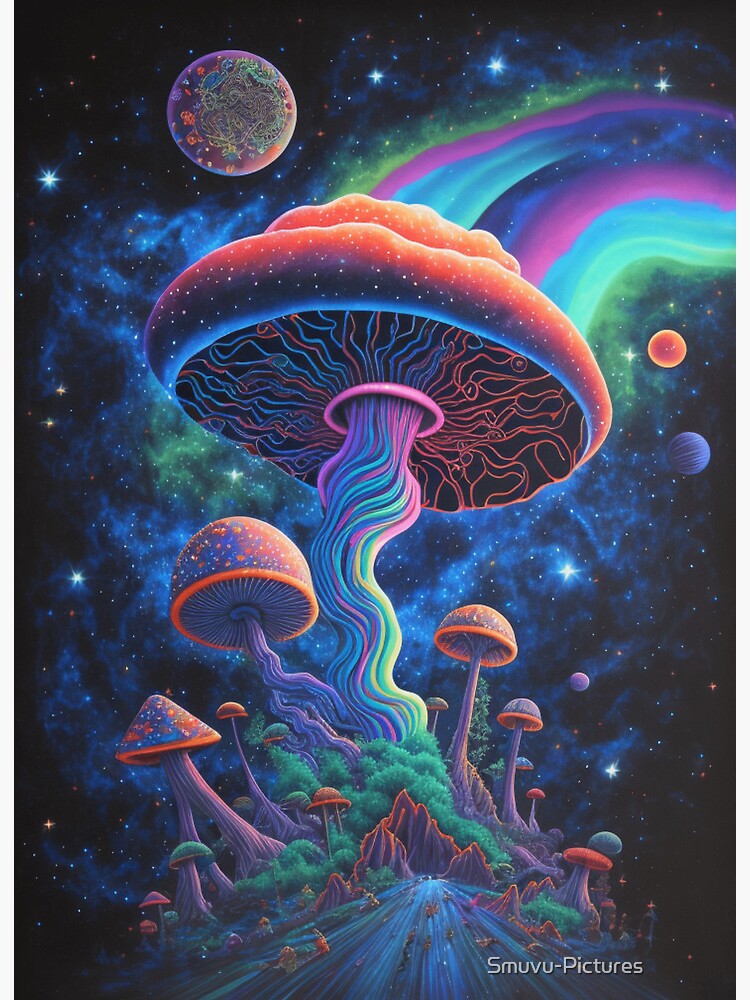The image features a vibrant and fantastical psychedelic artwork that captures the viewer's imagination with its vivid colors and surreal composition. Dominating the center is an enormous mushroom, reaching almost to the sky, with a reddish-orange canopy filled with small white dots and intricate, vein-like structures beneath it. Its stem brilliantly transitions through shades of blue, pink, and purple, creating a sense of movement and life. Surrounding the colossal mushroom are numerous smaller mushrooms sharing similar hues—orange caps with purple stems—sprouting amid trees, bushes, and gentle hillsides.

In the background, the night sky is a tapestry of colors with a black canvas dotted with stars in pinks, blues, and greens. The sky also features several planetary bodies and a multi-colored moon adorned with abstract art. A rainbow, composed of pink, blue, and purple bands, arches over the scene, further adding to its otherworldly charm. Below the majestic mushrooms, a winding road heads towards a distant mountain range, inviting viewers to journey deeper into this surreal landscape. The artwork is tagged with "SMUVU-Pictures," adding a touch of intrigue to the visionary scene.